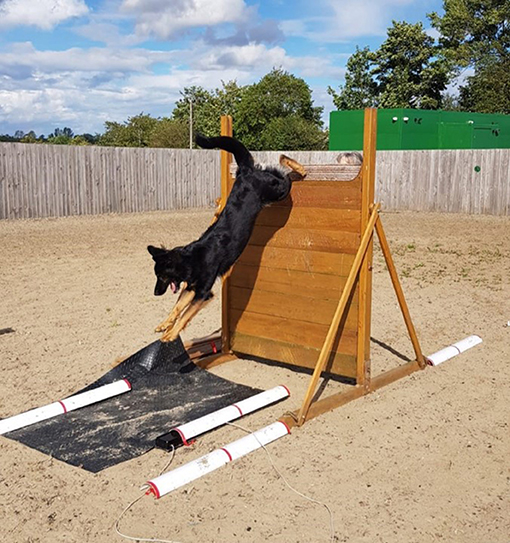This photograph captures a high-energy scene of a black and tan German Shepherd mid-jump over a wooden obstacle during what appears to be a competitive exercise. The dog's front legs, which are tan, are extended towards a black mat while its hind legs are still in the air. Its mouth is open, giving an impression of enthusiasm and excitement. The scene is set outdoors in a dry, gravelly yard enclosed by a wooden fence. In the background, behind the fence, there are green trees and a green building that resembles a shed. The sky above is filled with clouds. The wooden jump that the dog is clearing is surrounded by white panels and has strings or measuring implements attached to it. The attention to detail includes the presence of white weights that possibly support the structure. The atmosphere suggests a competitive or training environment, bringing out the agility and joyful spirit of the dog.